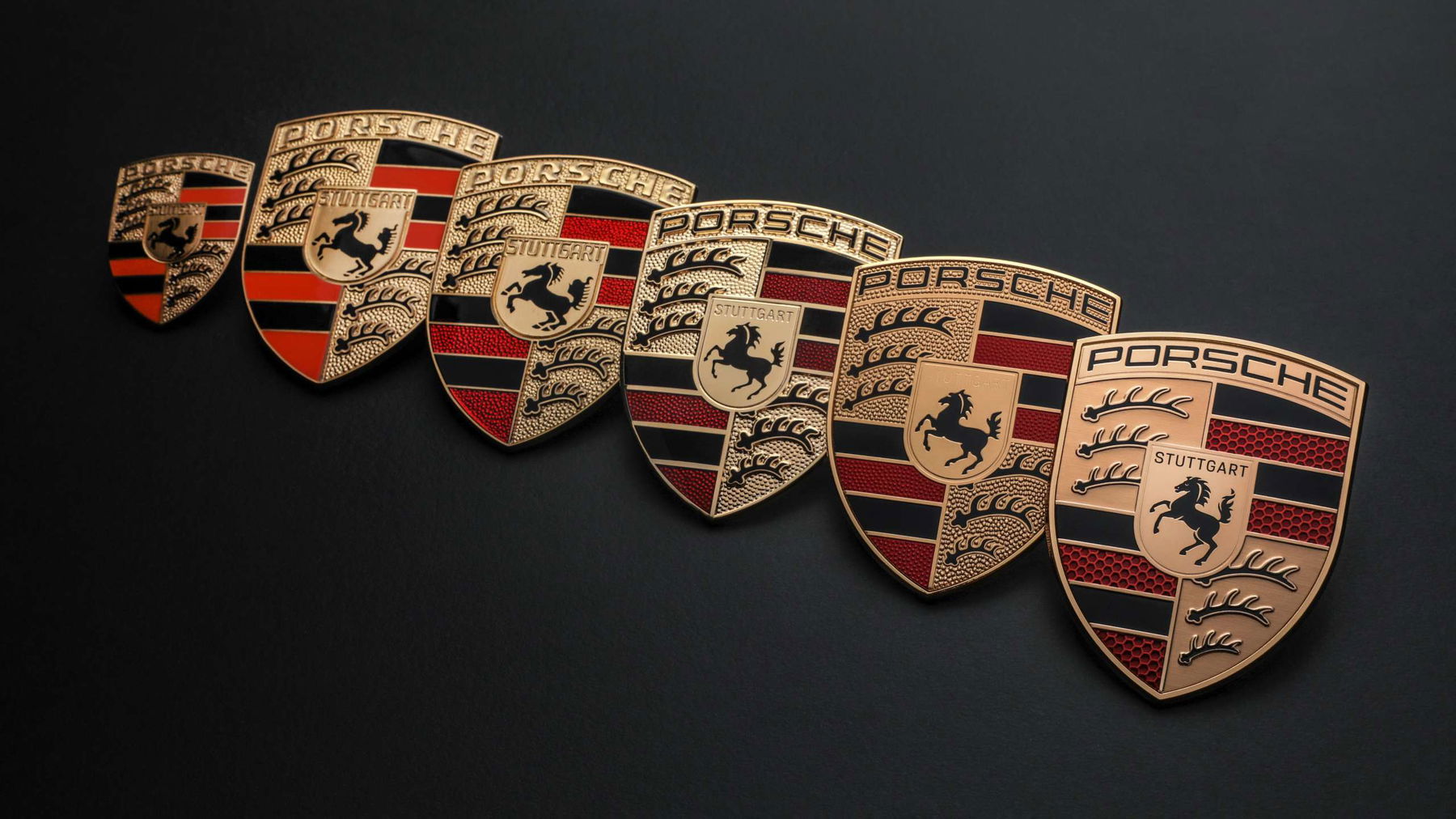The image depicts six Porsche emblems arranged in a line against a dark gray background. Each emblem is a shield, predominantly gold with detailed features. The top of each shield is emblazoned with the word "Porsche," with the first three logos featuring an embossed gold inscription and the last three showcasing black lettering. Centered on each shield is a black, rearing horse with its tail raised and front legs in the air, characteristic of Porsche's logo, and some emblems have the word "Stuttgart" written above the horse, varying between embossed gold and black. The logos are adorned with black and red stripes: black on the upper left and lower right, and red on the upper right and lower left of each shield. Each emblem also features intricate designs resembling antlers or ferns in the top left and bottom right sections. The smallest emblem is positioned at the far left, followed by five larger emblems, which are generally uniform in size but may have slight variations. The emblems appear metallic, reflecting the quality and detail associated with Porsche branding.